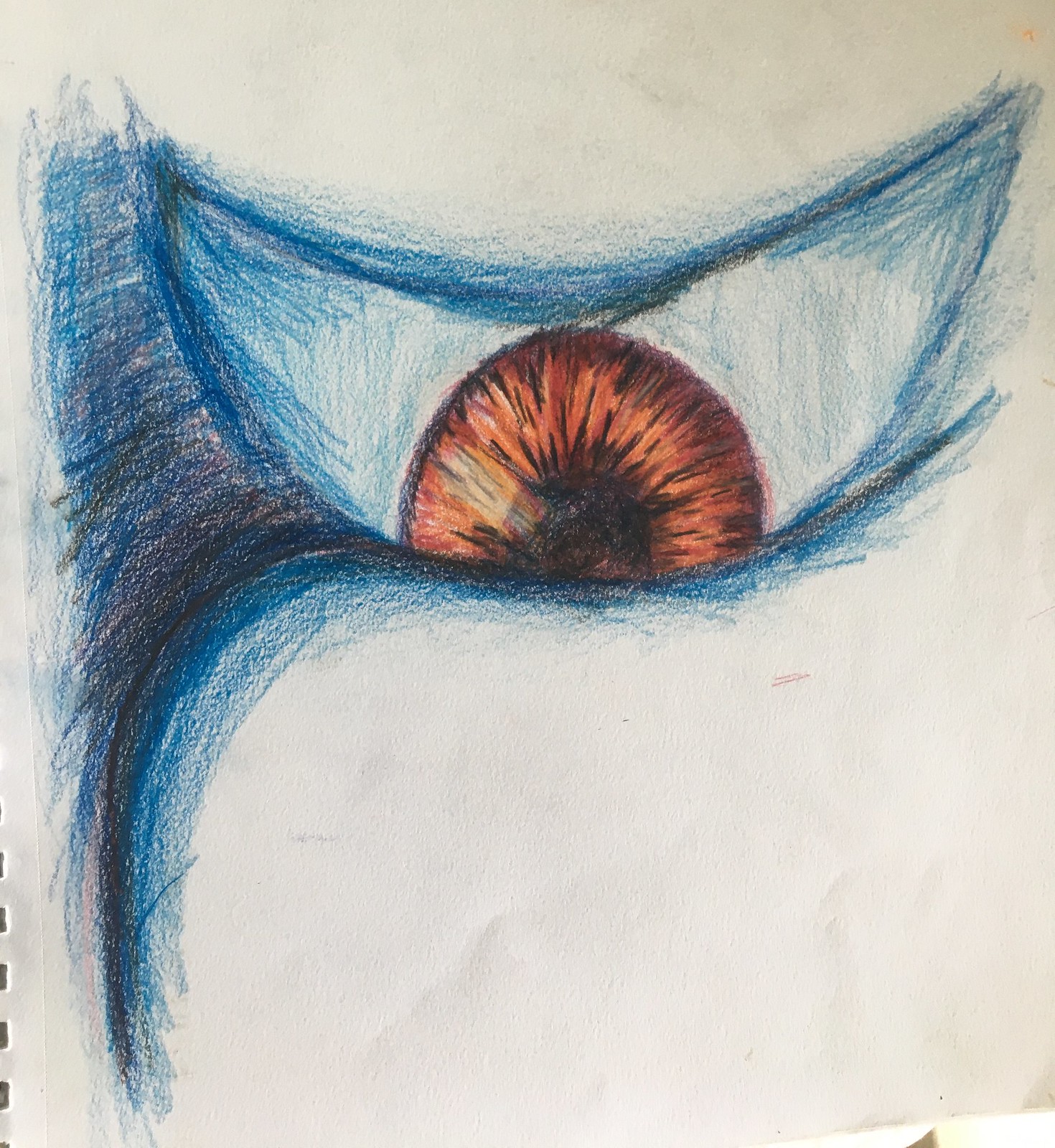This image captures a detailed sketch from a partially opened sketchbook, drawn with colored pencils. The drawing prominently features an eye, with an intricate iris centered around a large orange sphere encircled by a black border. Radiating from the center, black lines give texture and depth to the illustration, converging at the lower part of the eye into a solid black core. Surrounding the core is an upward-facing crescent half-circle, composed of vibrant blue lines edged with a hint of black, giving a dynamic and surreal effect. The drawing abruptly cuts off at the bottom, partially overlayed by more blue and black lines extending towards the left of the page. The bottom left corner of the image reveals the silver spiral bindings of the sketchbook, grounding the artwork within its physical medium.